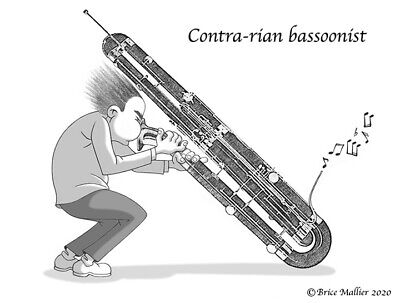In a detailed black-and-white illustration with a white background, a cartoonish depiction of a man energetically playing an oversized bassoon dominates the left side of the image. The man, slightly crouched and with bent knees, appears to be blowing intensely into the instrument—so much so that his hair is blown back, standing on end, and his cheeks are puffed out. The instrument, significantly larger than the man, rests on the floor with its body slanted toward him, emitting musical notes from its bottom end. Shadows of both the man and the instrument are visible beneath them, adding depth to the otherwise plain background. The man is clothed in trousers, a long-sleeved shirt, and shoes. In the upper right corner of the image, the text "Contrarian Bassoonist" is written in black. The lower right corner bears the black ink text "Copyright Bryce Miller 2020."